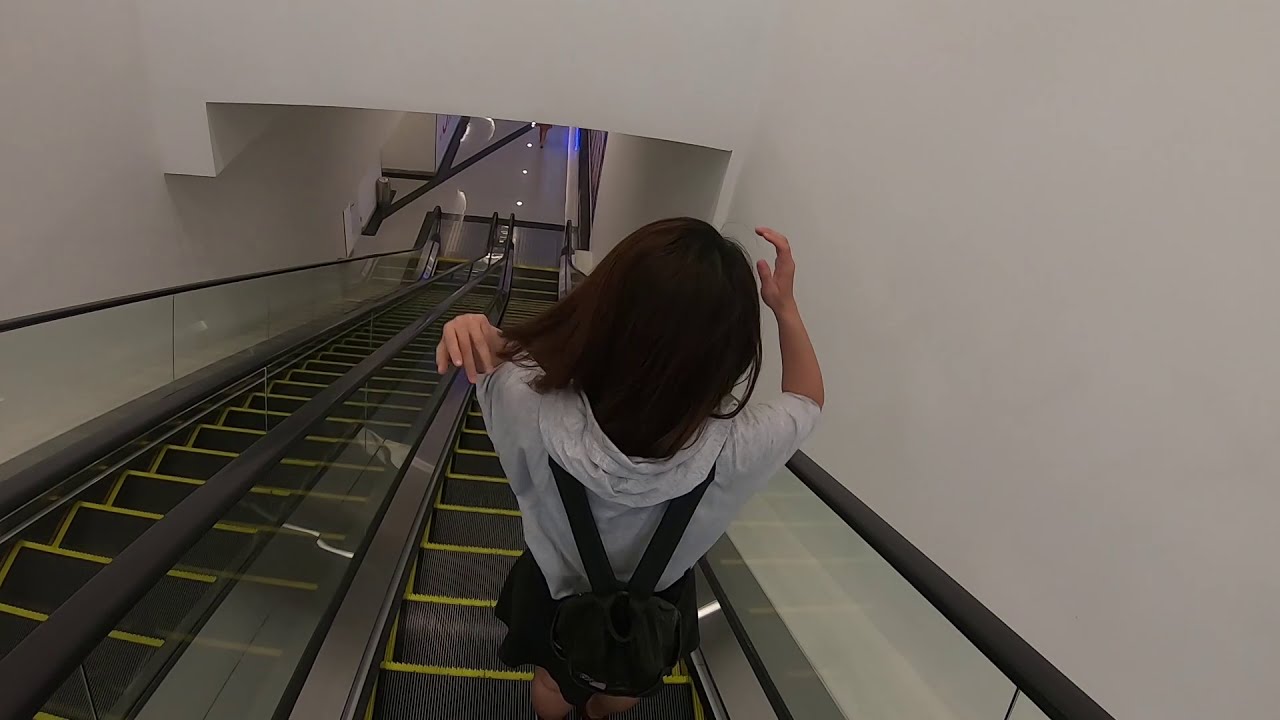The image captures a young woman descending a long escalator, her back to the camera. She is dressed in a light gray hoodie and a short black skirt, with a small black backpack slung over her shoulders. Her long dark hair, which falls to her shoulders, is being adjusted as she stands; one hand reaches up to the top of her head while the other brushes through her hair. The environment is stark and modern, featuring white walls and a white ceiling. The escalator itself has metal steps with yellow edges and black plastic rails. To her left is the ascending escalator. The setting transitions into an area below, characterized by minimal decor and punctuated with lines of white lighting on the floor, contributing to the clean, almost austere design.